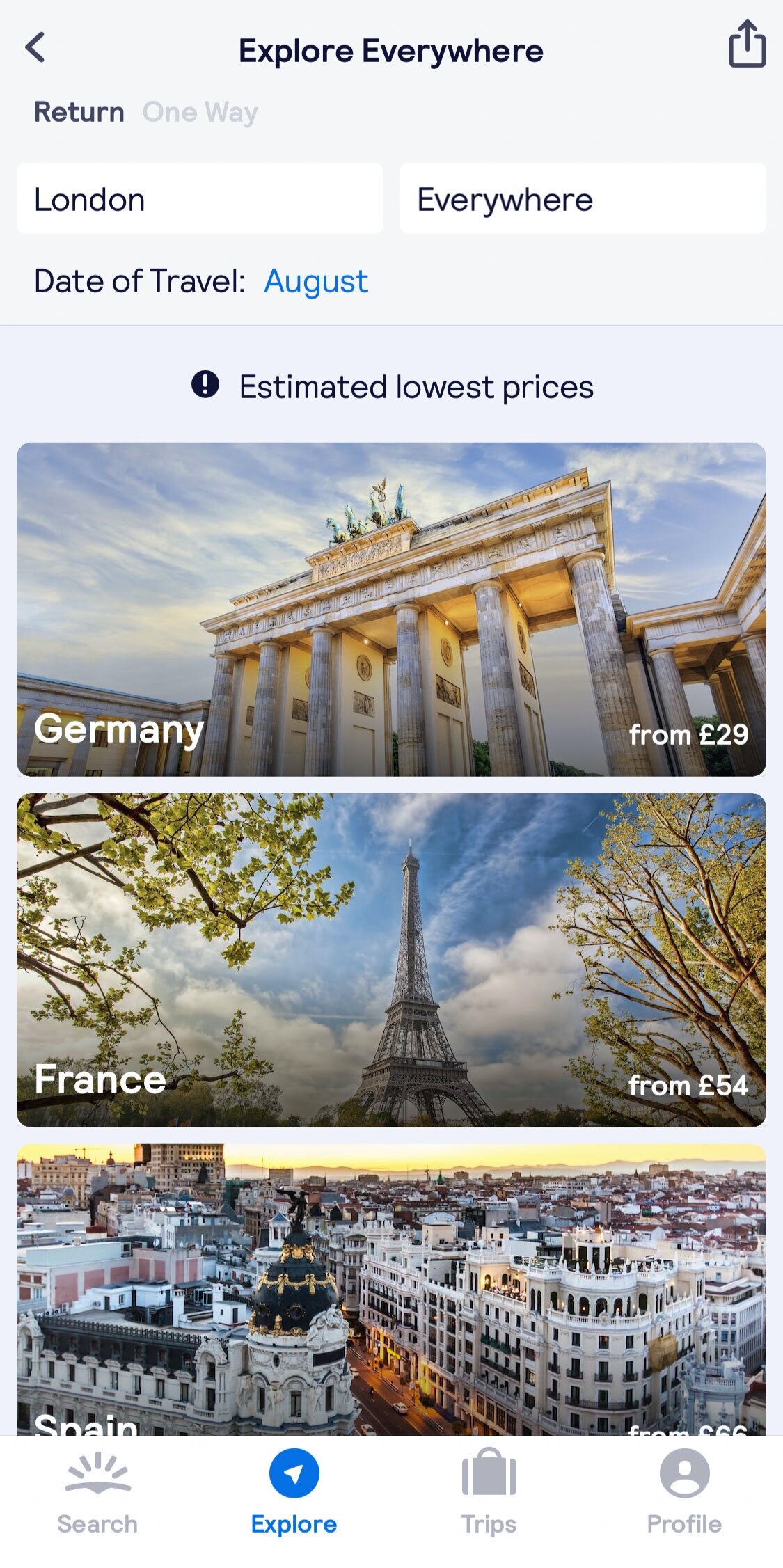The image displays a user interface from a travel-related app, likely on an iPhone, as indicated by the iPhone-styled download button. The background is predominantly white. At the center of the image, the phrase "Explore Everywhere" is prominently featured. Directly below it on the left side, options for "Return" and "One Way" travel are available. Underneath these options, two white input boxes show "London" and "Everywhere" respectively. Beneath this, the text "Date of Travel: August" is displayed.

The bottom portion of the interface features three destination images with estimated lowest prices. Each image includes a small exclamation point icon and the phrase "Estimated Lowest Prices" in the center of the image.
 
1. **Germany**: The first image at the top showcases a large, historically significant building in Germany, perhaps a landmark or a capitol building, set against a clear, daytime sky. "Germany" is written in white letters at the bottom of the image, and to the right, text indicates prices starting "from 29 GBP".

2. **France**: The second image features the iconic Eiffel Tower in France, taken during the daytime with visible blue skies and surrounding greenery. The word "France" appears in the picture with a price indication "from 54 GBP" at the right.

3. **Spain**: The final image displays a picturesque view of what appears to be a densely built area of Spain, possibly Madrid. With a sunrise or sunset adding a warm glow, the area looks vibrant, featuring numerous buildings and possibly some hotels and a capitol dome. The text "Spain" is written, with prices starting "from 66 GBP" to the right.

At the bottom of the interface, navigational buttons for "Search," "Explore," "Trips," and "Profile" are visible, completing the intuitive user layout of the app.

Overall, the image effectively presents visual and textual information aimed at assisting users in exploring and booking travel destinations with ease.